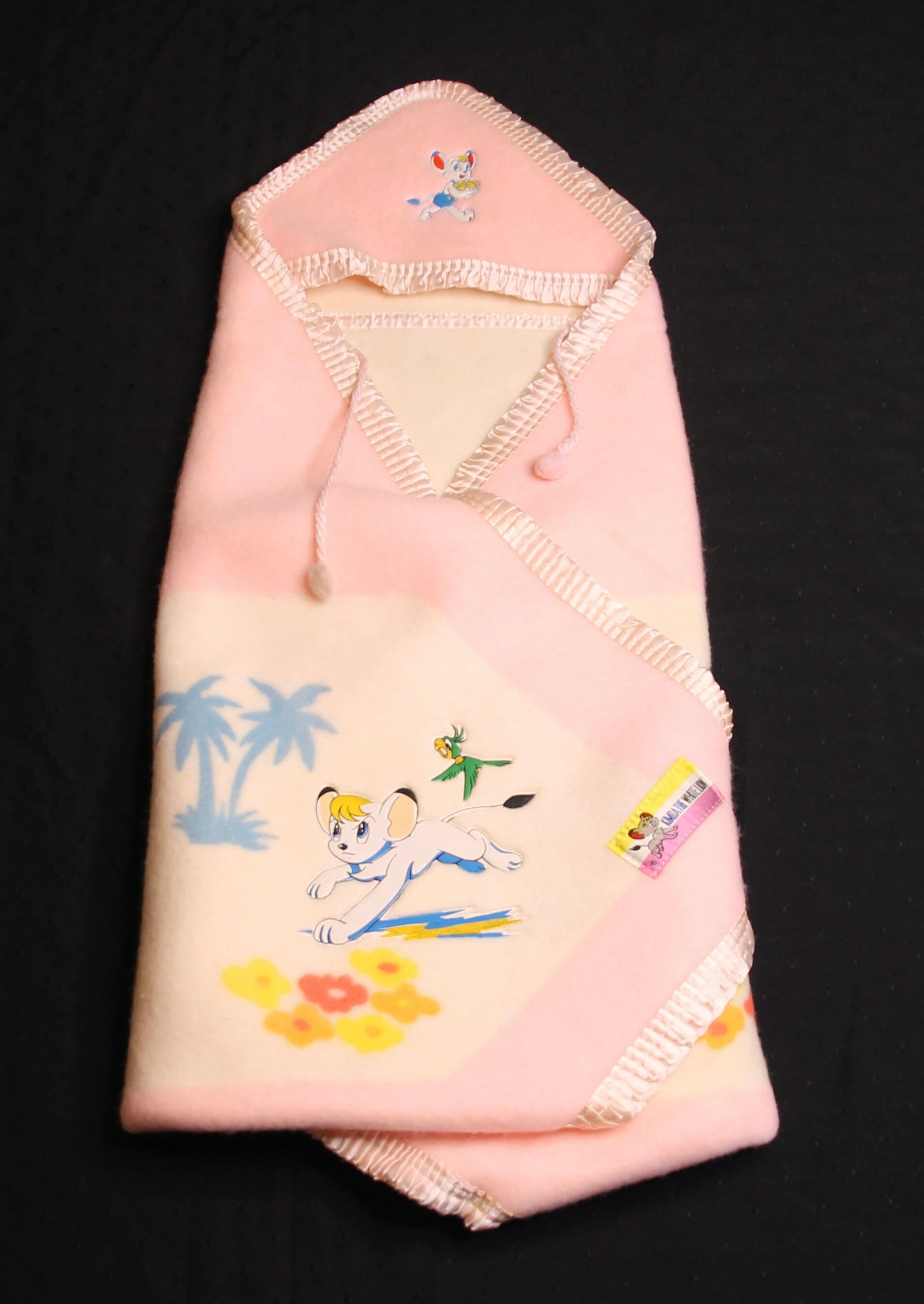The image depicts a small cloth item, possibly a custom-made infant bib or shirt, designed with a pink background and pink strings for neck ties. The fabric is adorned with vibrant yellow, orange, and red flower petals on one section. A whimsical cartoon character, likely a mouse with blue and white fur and yellow hair, adds to the playful design. Alongside the mouse, a green bird with a yellow beak is also featured, as well as blue palm trees that create an exotic setting. The item appears to be photographed on a black surface, perhaps for display purposes. A blurred tag is present, although its details are not discernible. The overall pattern and colors, along with the folded triangular section, suggest it's ideally suited for a newborn, exuding a cute and charming aesthetic.